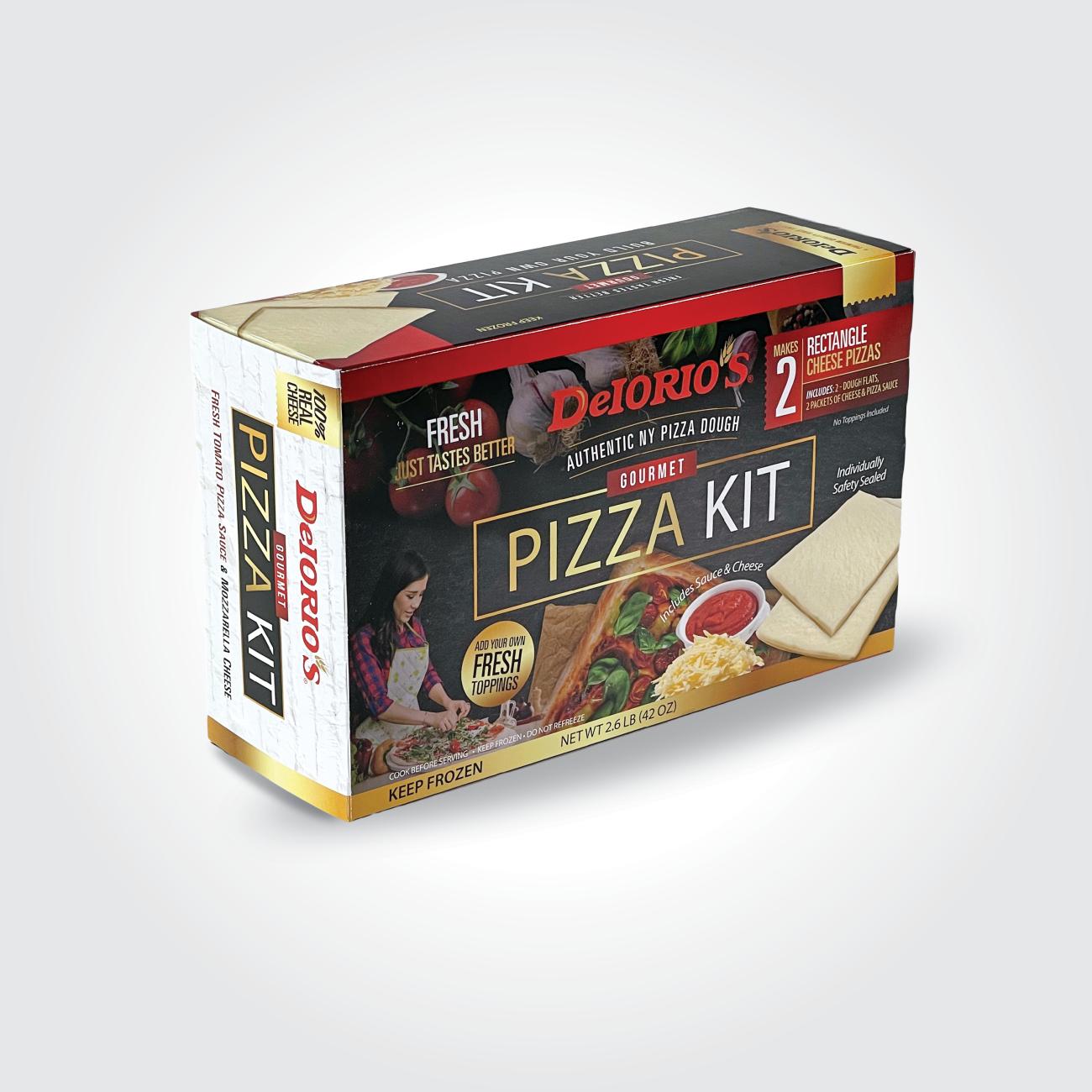Featured in this professionally edited product photograph is a gourmet pizza kit from the brand D-E-Oreos, packaged inside a rectangular cardboard box. The box appears to be suspended in an empty white void with a subtle shadow added underneath for depth, giving a clean and appealing presentation. The image is taken at an angle allowing a view of the front, top, and left sides of the box. The front of the box prominently displays the brand name and product description: "Authentic New York Pizza Dough - Fresh, Just Tastes Better. Add Your Own Fresh Toppings." The kit includes dough, sauce, and cheese, allowing you to create your own pizza by adding fresh toppings.

In addition, there is detailed imagery and text on the box, which calls out that the kit makes two rectangular cheese pizzas, with ingredients safely sealed for freshness. The visual elements include vibrant colors such as white, red, gold, black, pink, purple, and green. Illustrations depict tomatoes, onions, shredded cheese, sauce, and a pizza to suggest the variety of toppings you can add. The box also features an image of a woman in an apron spreading toppings over a round pizza, emphasizing the hands-on, customizable aspect of the product.